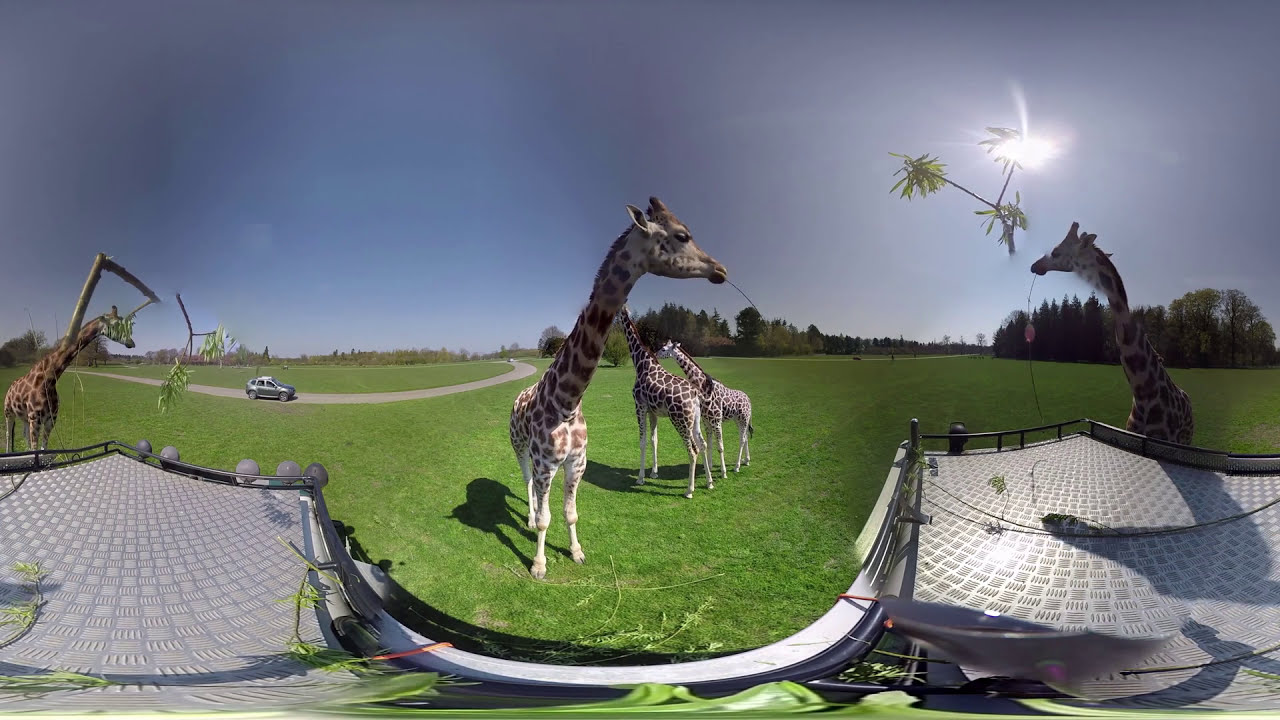This captivating 360-degree panoramic image transports us to an animal sanctuary, capturing a picturesque scene bathed in bright, sunny daylight with a clear blue sky. At the center of the composition are six giraffes, their distinctive necks seemingly even longer due to the panoramic distortion. The giraffe nearest to the viewer has its neck extending directly towards us, emphasizing the intriguing visual twist. The animals, including both adult and juvenile giraffes, are in a large, meticulously maintained grassy field.

Against this verdant backdrop, there's a gray stone or tile viewing platform with a protective fence, allowing visitors a safe vantage point without the risk of falling. In the background, a small road meanders away from the field, with a car visible that hints at the sanctuary's drive-through feature for wildlife observation.

Artifacts from the panoramic stitching lend an ethereal quality to the sky, where bits of vegetation seem oddly placed. To the left, elements suggesting the top of a safari vehicle, including fog lights, anchor the scene, reiterating the adventure of wildlife observation. This sanctuary, lush and well-tended, offers a gentle reminder of the efforts to create safe havens for these majestic creatures.